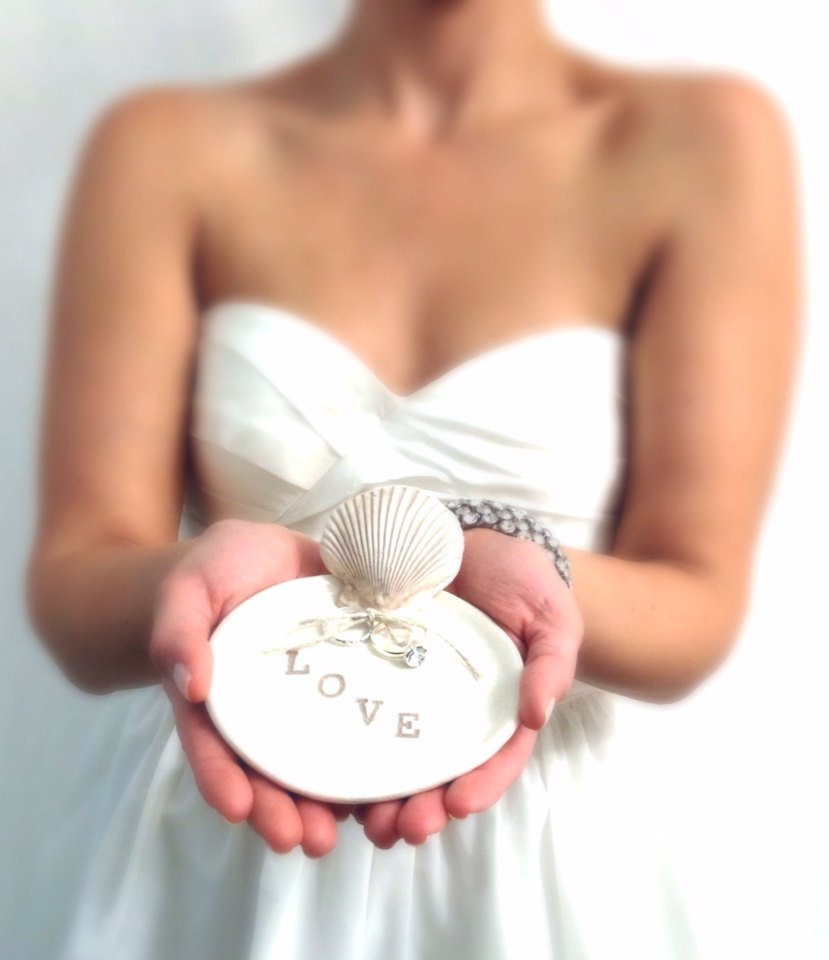In this photograph, a Caucasian woman is depicted from her torso down, dressed in a white, sleeveless bridal gown with a wraparound style that reveals her arms and the top of her chest. Her manicured hands, devoid of nail polish, are prominently positioned towards the camera. In her left hand, adorned with a silver bracelet embellished with what seems to be diamonds or rocks, she holds an intricately designed decorative plate. This circular plate bears the word "LOVE" arranged diagonally from top left to bottom right, with a seashell affixed to its top part. Attached to the seashell is a string or twine, which holds two rings—a man's and a woman's engagement or wedding ring—dangling at the center. The photograph is taken in a style that focuses on these elements, with a somewhat blown-out white background that makes the intricate details of the plate stand out vividly. The absence of the woman's head in the image places more emphasis on the gown and the meaningful object she holds.